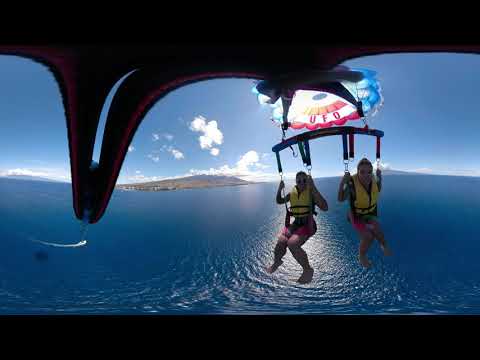In this captivating outdoor photograph set on a brilliantly sunny summer day, the scene unfolds with deep, serene blue ocean waters and a nearly cloudless, bright blue sky dotted with a few light, fluffy clouds. The horizontally rectangular image is framed with black borders at the top and bottom, adding to its panoramic feel. Central to the composition is a stretch of land that rises slightly from the water, perhaps an island set in the distance.

Dominating the scene are two girls engaged in a thrilling parasailing adventure. Suspended side by side on harnesses, their attire is strikingly identical: they wear pink shorts, yellow life jackets, and sunglasses, their legs barefoot and legs openly visible. Above them, a vibrant red, white, and blue parasail catches the eye, emblazoned with the word "UFO." This sail has blue and red edges with a white midsection, creating a bold visual contrast against the sky. The girls appear to be firmly gripping their harnesses, adding a tangible sense of adventure and excitement to the image.

The picture gives the impression of being captured from a unique perspective, possibly the reflection of a rearview mirror, which adds an intriguing, almost voyeuristic element. The distant landmass on the left adds depth and context to their high-flying adventure. This snapshot of parasailing captures the essence of summer fun and the exhilarating freedom of soaring above the vast ocean expanse.